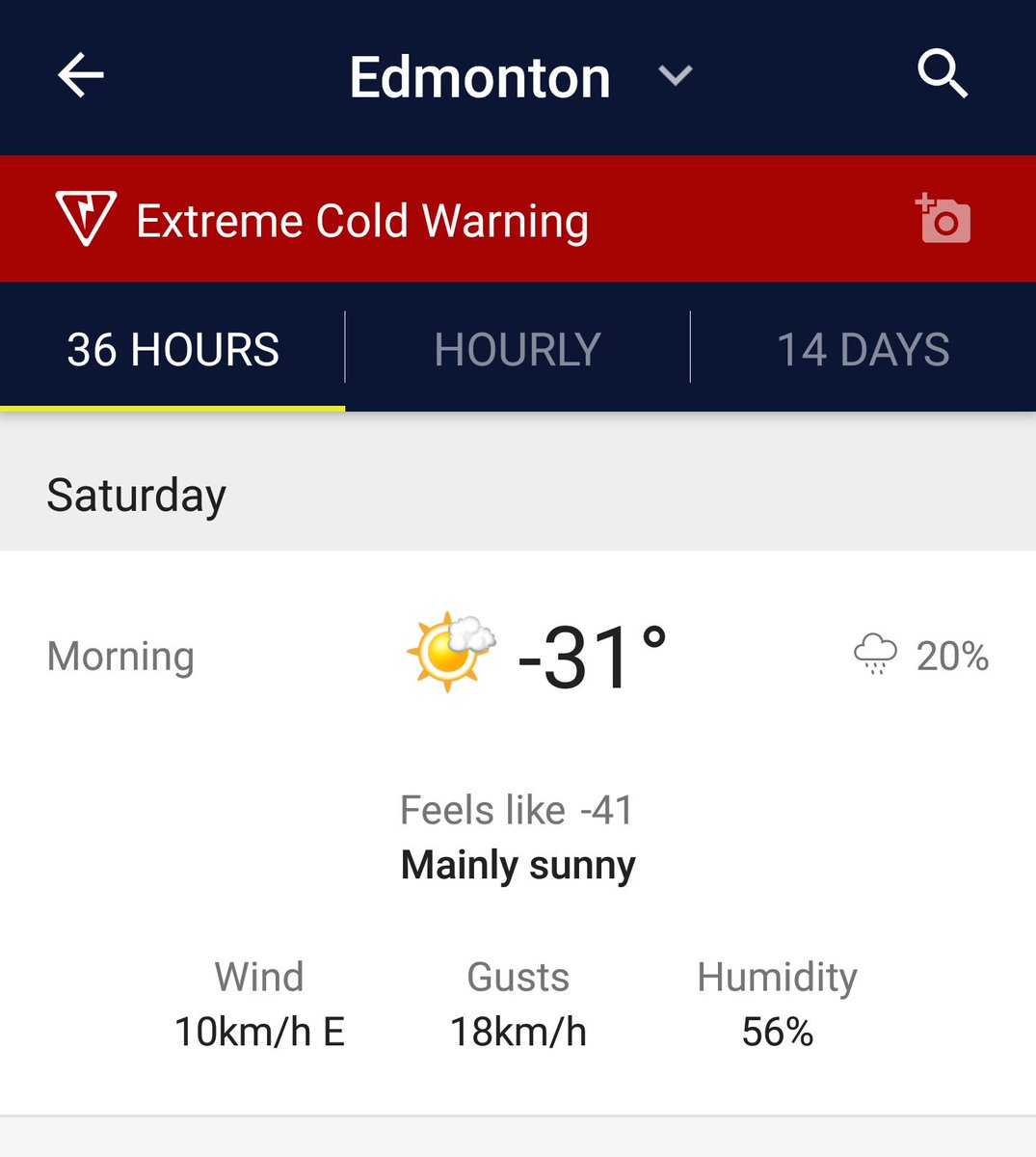The image starts at the top with a navy blue section. A white arrow pointing left is displayed on the left-hand side. In the center, "Edmonton" is written in bold white font. A small down arrow, resembling half a triangle, is present below the text. On the right-hand side, a magnifying glass icon is also in bold white.

The next horizontal section is red. In white font, a triangle with a lightning bolt-like design inside it is present. Beside it, "Extreme Cold Warning" is written in white. A small icon is situated on the far right.

The following section is another rectangular navy blue area. On the left, "36 HOURS" is written in bold white uppercase letters, followed by a light vertical line. "HOURLY" is next, also in uppercase. Another vertical white line precedes "14 DAYS," again in bold uppercase letters. The "36 HOURS" text is underlined with a fluorescent or neon yellow line.

Below this, on an off-white background, "Saturday" is written in bold black font. "Morning" is listed in regular black font on a white background. In the middle, an icon of a sun partially covered by a cloud in the upper right is present. Next to it, the temperature is marked as "-31°C" in bold black font. To the right, a cloud icon with raindrops and "20%" is displayed. Under "-31°C," the text "Feels like -41" is written in regular black font.

Additionally, "Mainly Sunny" is noted in bold font. Beneath this, aligned slightly to the left, "Wind" is written in regular black font. Next to it, in bold, it reads "10 km/h E." The next column states "Gusts" in regular font with "18 km/h" bolded beneath it. The third column mentions "Humidity" with "56%" bolded below. 

Finally, a horizontal rectangular box stretches across the bottom of the image.